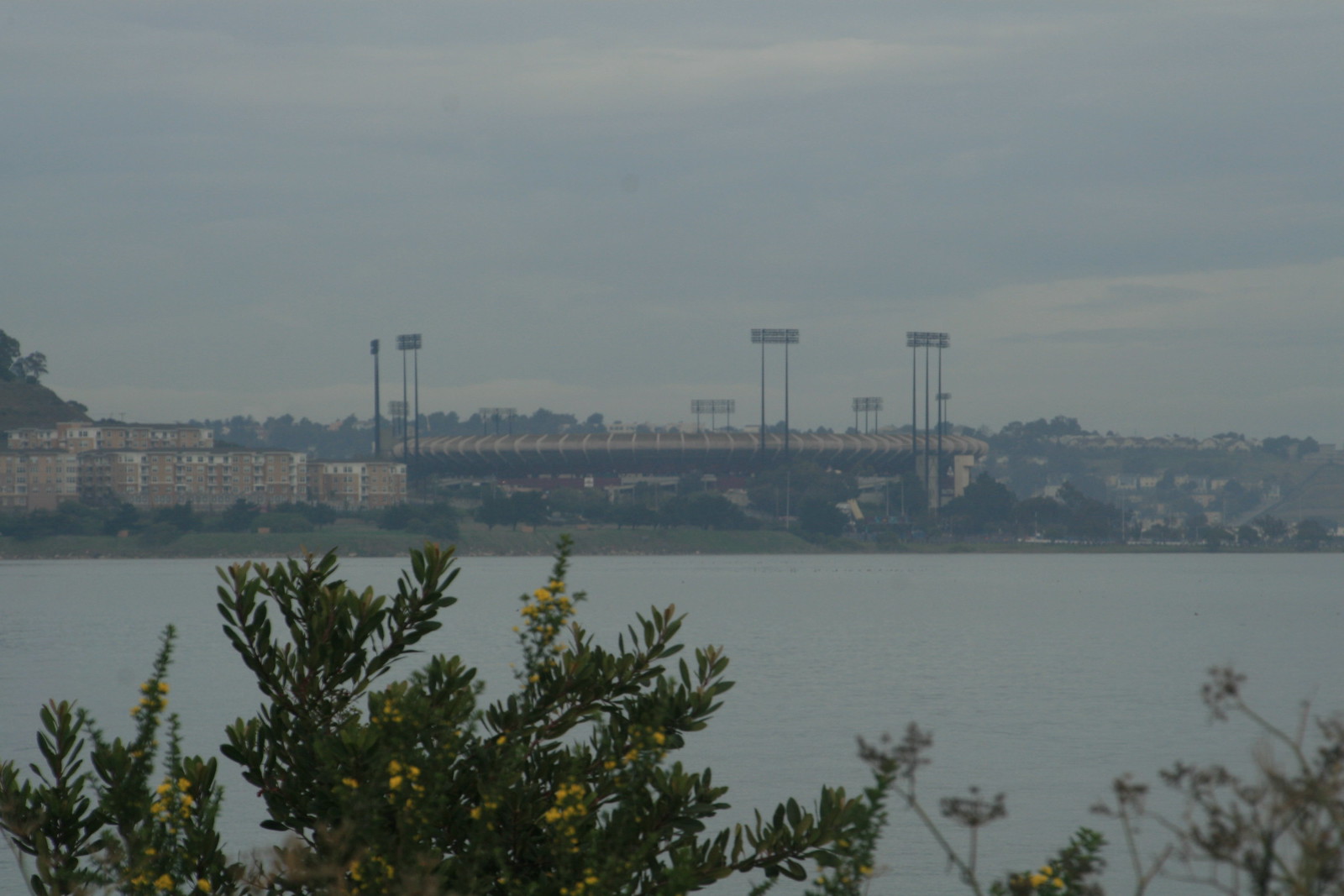The image depicts a foggy, grayish-white sky over a calm, grayish-blue river. In the foreground, small green shrubs with green leaves and yellow flowers line the riverbank. Across the river, on the left, there's a cluster of residential buildings, distinguishable by their brown and white exteriors and dark roofs. To the right of these buildings is a structure resembling a tunnel-like bridge, covered and marked with white lines, surrounded by several tall stands. This structure appears to be part of an outdoor stadium, possibly the Oakland Coliseum, given its dated, spaceship-like appearance and the numerous high spotlights that would illuminate it at night. The entire scene is enveloped in a misty haze, adding a serene yet mysterious ambiance.